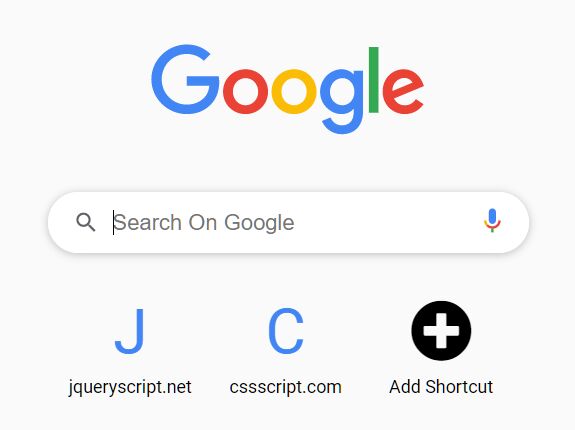The image is a screenshot with a gray background featuring the Google homepage. Prominently displayed is the Google logo, with the letters "G", "o", "o", "g", "l", and "e" in blue, red, yellow, blue, green, and red, respectively. Below the logo, there's a search bar with the placeholder text "Search on Google." 

A blinking cursor is positioned at the beginning of the search bar text. To the left of the search bar is a microphone icon, and to the right is a magnifying glass icon, representing the search function. Additionally, below the search bar, there are two links displayed: 

- The first is "jqueryscript.net" next to a blue "J".
- The second is "cssscript.com" next to a blue "C".

Finally, a black circle featuring a white plus sign and ellipsis is positioned near the bottom, accompanied by the text "Shortcut."